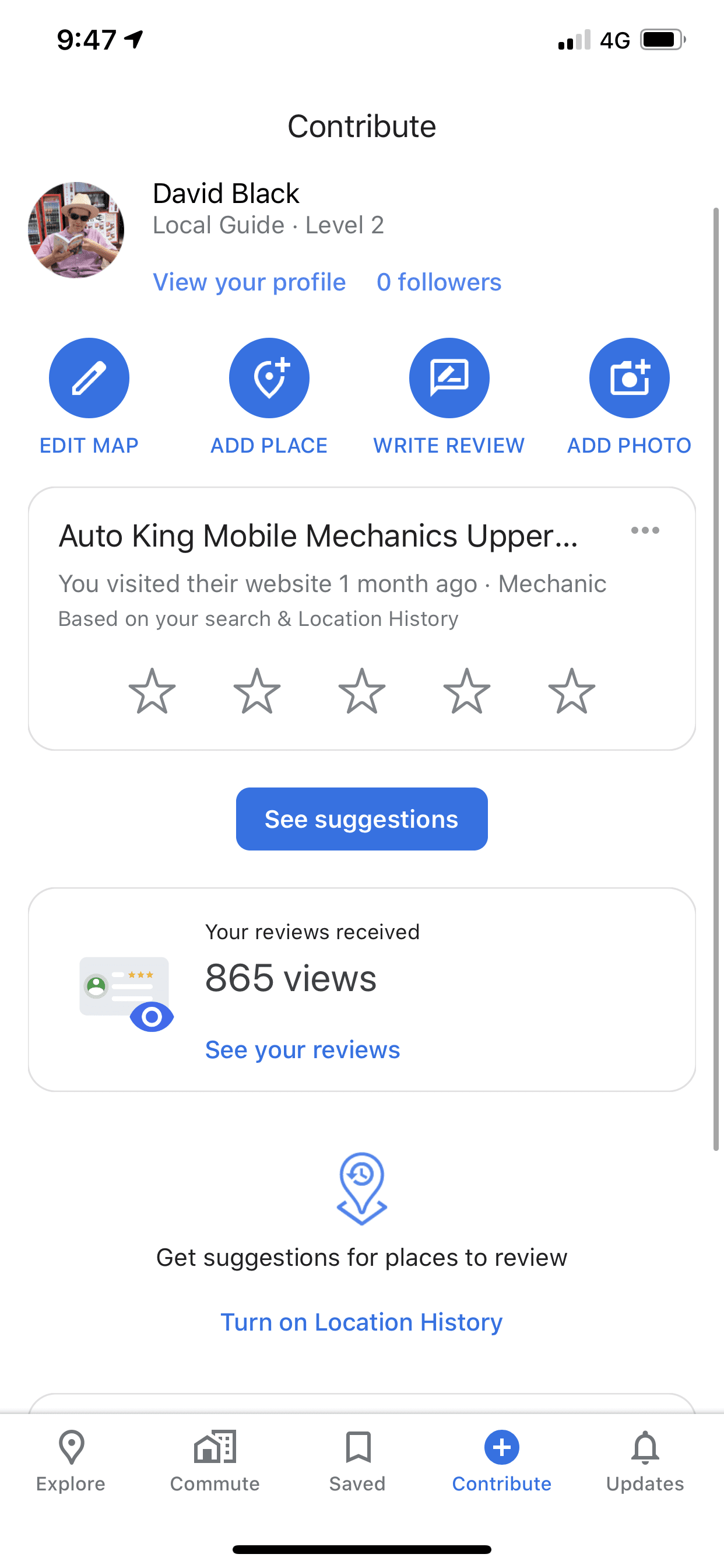In this image, we see a screenshot from a mobile device. In the upper left corner, black text indicates the time as 9:47. The upper right corner displays icons for the battery level and 4G connectivity. 

The main content of the screenshot is centered against a white background. At the top, the text "Contribute" is prominently displayed. Below this, there is a profile for a user named David Black. The profile includes an image of a man wearing sunglasses and a hat, reading a book. Under David Black's name, grey text reads "Local Guide Level 2." 

Beneath this profile, there are four blue circular icons from left to right labeled: "Edit Map," "Add Place," "Write Review," and "Add Photo."

Below these icons, "Auto King Mobile Mechanics" is written in black text. Under this, light grey text mentions, "You visited their website one month ago," followed by, "Mechanic, based on your search and location history." At the bottom of the image, there is a blue button labeled "See Suggestion."